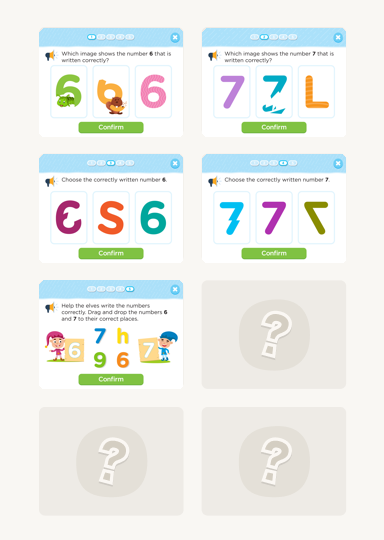The image depicts a vertically-oriented gray box segmented into multiple smaller boxes. Each smaller box has a blue top and contains a combination of numbers and letters, typically three per box. 

**First Smaller Box:** Displays a green "6", an inverted "A"-like shape, and another green "6". The background colors are green and yellow, with a small monkey illustration in the middle and a green bug image next to one of the green sixes.

**Second Smaller Box:** Contains the sequence "77L" with the first "7" in purple, the second "7" in blue, and the "L" in orange.

**Third Smaller Box:** Features a "C" in dark maroon, an "S" in orange, and a "6" in green.

**Fourth Smaller Box:** Shows two "7"s in teal and purple, followed by a backward "7" in a darker shade of green.

**Fifth Smaller Box:** Highlights two cartoon characters; the character on the left is holding a "6", and the one on the right is holding a "7", both colored in yellow. Also, it includes a blue "7", a yellow "H", a green "9", and an orange "6".

Beneath these smaller boxes, there is a green button labeled "Confirm" for validation. The accompanying instructions, located above the gray box, prompt the viewer to identify numbers, such as matching the correctly written number "6". Three of the smaller boxes feature question marks enclosed in circles, indicating areas requiring attention or further interaction.

The overall image appears to be an educational tool or a learning activity designed to help users recognize and differentiate numbers and letters, possibly in a playful context with engaging visual elements, such as the cartoon characters and the monkey illustration.